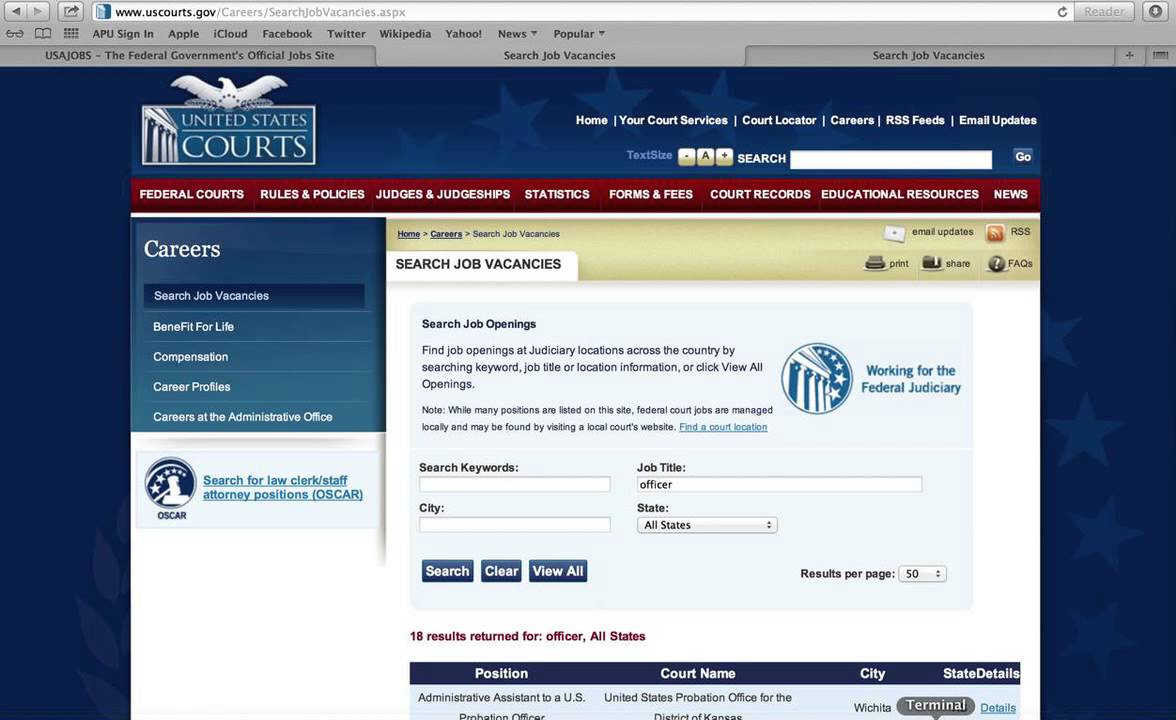The United States Courts website features a comprehensive navigation menu set against a navy blue background. The menu includes options such as "Home," "Your Court Services," "Court Locator," "Careers," "RSS," and "Email Updates." Positioned prominently above the menu is the website's emblem, an eagle symbolizing the federal judiciary.

To the side, there's a striking image of a section of the Supreme Court building, adding a touch of gravitas to the page. Overlaying this background is a red banner section that provides quick access to various important links, including "Federal Courts," "Rules and Policies," "Judges and Judgeships," "Statistics," "Forms," "Feeds," "Court Records," "Educational Resources," and "News."

The careers section is particularly detailed, enabling users to search for job vacancies at judiciary locations nationwide. Users can filter job openings by keywords, job titles, or specific locations, or they can click "View All Openings" to see a comprehensive list. It is important to note that while many job positions are listed on this website, actual hiring is managed locally, necessitating visits to individual court websites for more details. A link to find local court websites is highlighted in teal.

For instance, in one job search example, a user looking for "officer" positions across any location in the United States returned 18 results, with an option to display 50 results per page. 

This provides a snapshot of the robust resources available on the United States Courts website, though the site contains significantly more information and services beyond the section described.